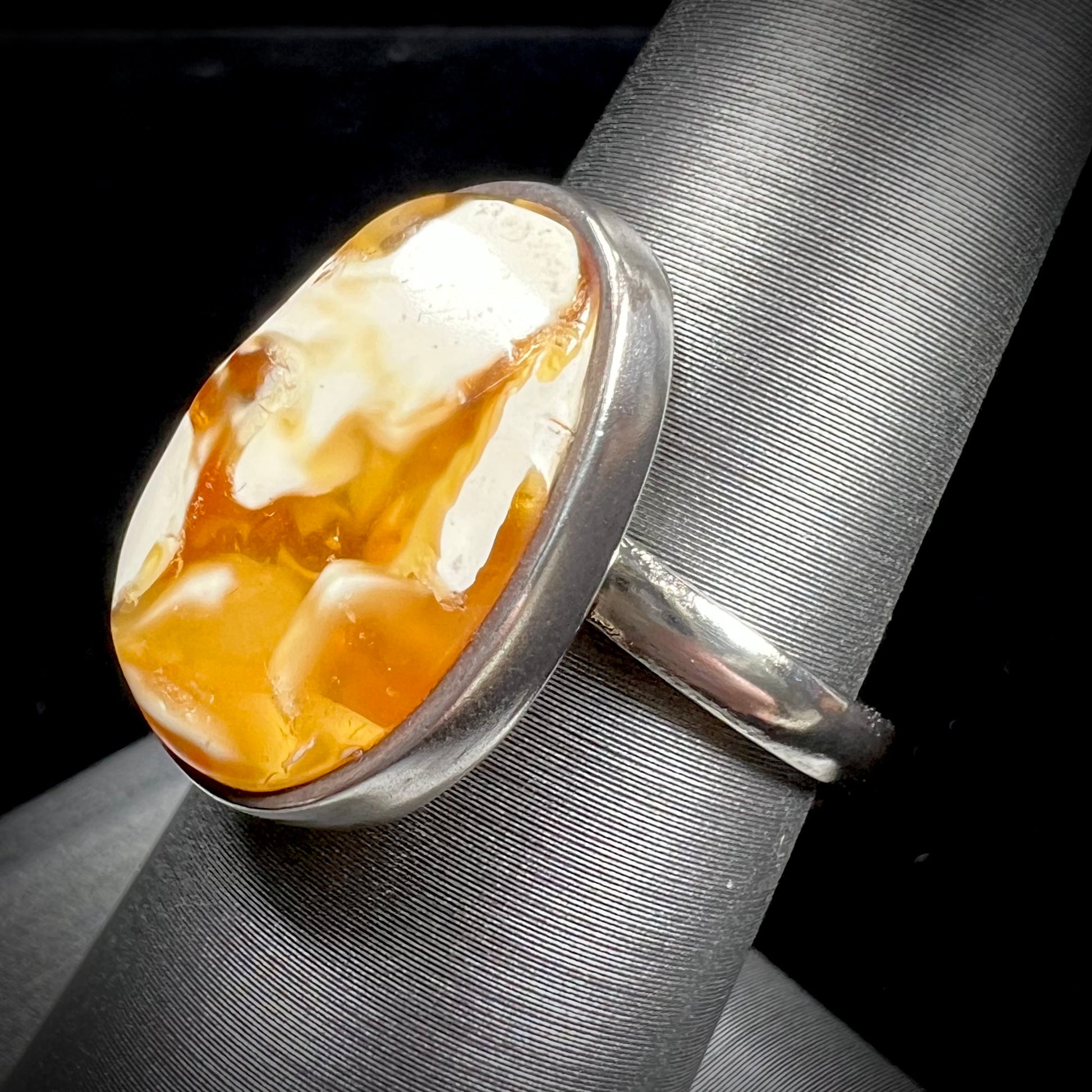In a vertical rectangular photograph set against a stark black background, a large, ornate ring is prominently displayed. The ring is mounted on a textured silver cylinder designed to resemble a finger. The band of the ring is thick and silver, matching the color of the mounting pole which features textured rivets and culminates in a silver square base at the bottom. The centerpiece of the ring is an oval-shaped stone that draws immediate attention with its rich color gradient. The stone transitions from bright white at the top edges to a deep royal brown towards the bottom, accented by a small white stripe. The vibrant, gem-like appearance of the stone contrasts sharply with the monochromatic, metallic setting of the silver band and background elements, making the ring's intricate details and colors pop dramatically in the image.